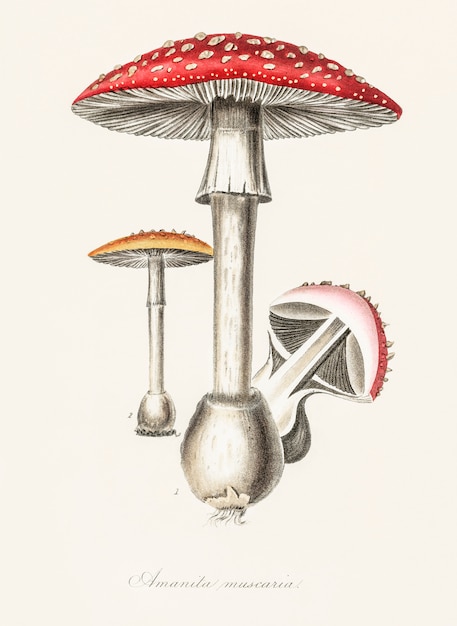The image depicts a meticulously hand-drawn illustration of three distinct mushrooms on a beige background, which might be from a magazine or a book page. At the center of the illustration is a prominent mushroom characterized by a long, white stem with a flared base, topped with a red cap adorned with white flakes. To the left, in the distance, stands another mushroom with a thin white stem, an orange, oval-shaped cap, and a flared base. The mushroom on the right leans at an angle, showcasing its underside, which is pink-topped with a white cylindrical stem. Underneath these detailed illustrations, there is faint cursive text believed to read "Amanita Muscaria." The overall art is well-preserved and elaborately detailed, with black borders accentuating different parts, indicating it may be an older but well-maintained piece.